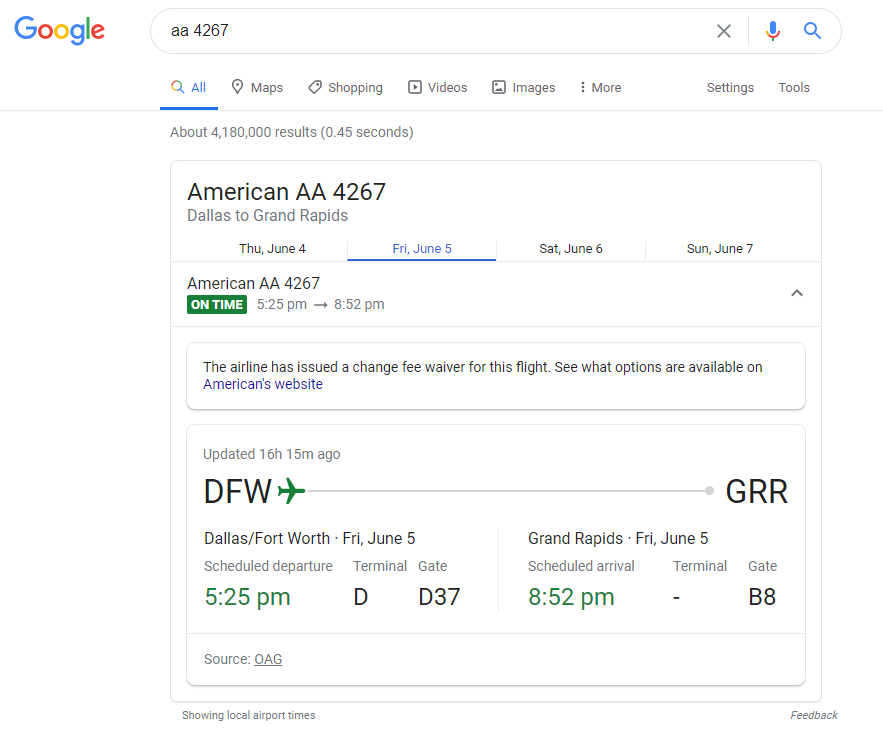Screenshot showcasing a Google search result for the flight number AA4267. The search bar at the top prominently displays "AA4267". The first search result provides detailed information about American Airlines flight AA4267, traveling from Dallas to Grand Rapids. Below the primary result, various tabs list dates: Thursday, June 4th, Friday, June 5th, Saturday, June 6th, and Sunday, June 7th. The highlighted information shows that flight AA4267 is scheduled to depart on time on Friday, June 5th, with a flight duration from 5:25 PM to 8:52 PM. There is a note indicating that the airline has issued a change fee waiver for this flight, with options available on the American Airlines website. The update timestamp reads "16 hours 15 minutes ago". The departure point, Dallas/Fort Worth International Airport (DFW), is on the left side, and the arrival point, Gerald R. Ford International Airport (GRR) in Grand Rapids, is on the right. Specific details include a scheduled departure from Terminal D, Gate D37 at DFW and a scheduled arrival at Gate B8 at GRR on Friday, June 5th.